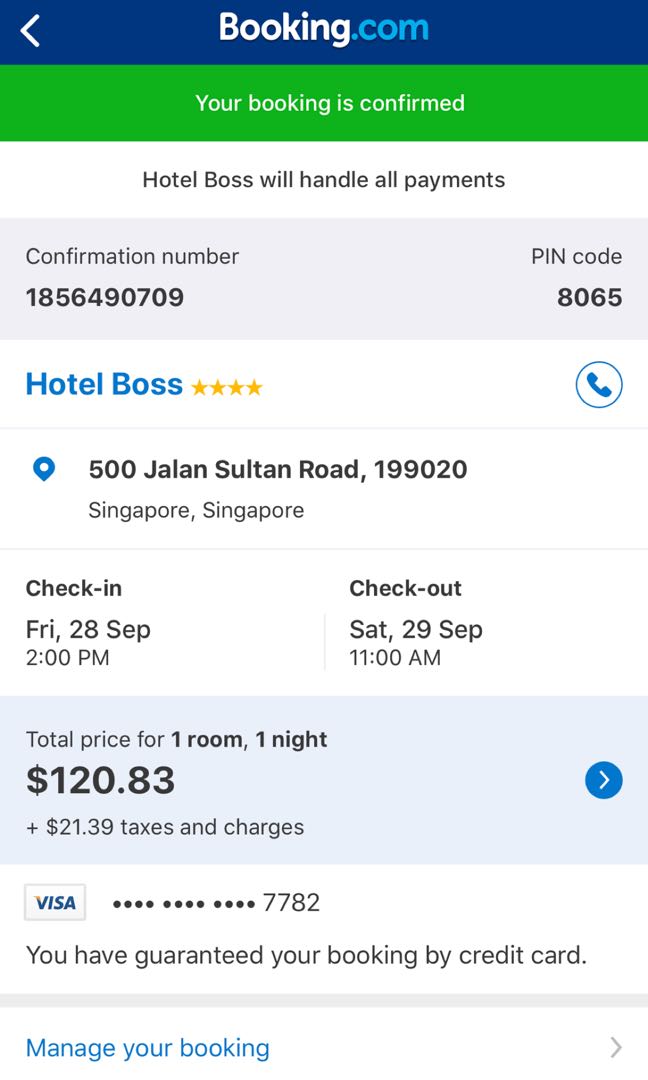**Website Booking Confirmation Overview**

At the top of the website is a dark blue header with the label "Bookings" in white text, accompanied by "booking.com" where the ".com" is highlighted in blue. A white left-facing arrow is also present on this dark blue strip.

Below, a green band displays a confirmation message in white text: "Your booking is confirmed."

Further down, on a gray band, additional details are provided: 

- Hotel: "Hotel Boss" (4 stars)
- Confirmation Number: 1856490709
- PIN Code: 8065
- Address: 500 Julianne Sultan, Sultan Road, 199020, Singapore, Singapore
- Check-in: Friday, 28 September at 2:00 PM
- Check-out: Saturday, 29 September at 11:00 AM
- Total Price: 1 room, 1 night, $120.83 plus $21.39 in taxes and charges
- Payment Method: Visa, ending in 7782

A blue circular button with a white phone icon allows users to call the hotel directly.

At the bottom, a blue button marked "Manage your booking" with a right-facing arrow helps users modify their reservations. Similarly, on the pricing section, a blue arrow on a gray background indicates further navigation options.